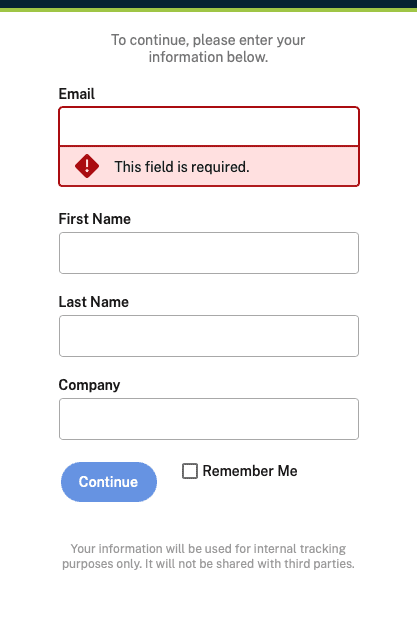Screenshot of a login page featuring a distinct header with black and green stripes merged together. Below the header, centered at the top, is the prompt "To continue, please enter your information below." The page contains four input fields arranged in a vertical format:

1. **Email:** The input box for typing in an email address is outlined in red, indicating an error. Inside the box, there's a light red shading, and just beneath it, a small red banner states, "This field is required."
2. **First Name:** This box is currently empty.
3. **Last Name:** This box is also empty.
4. **Company:** This input field is empty as well.

Beneath the "Company" field, there is a blue "Continue" button and a checkbox labeled "Remember me." Below these elements, gray text notes that "Your information will be used for internal tracking purposes only. It will not be shared with third parties." The entire form is set against a white background.